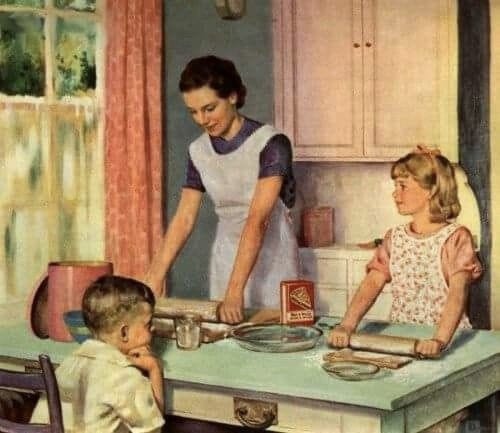The image depicts an old-fashioned, likely mid-20th-century illustration of a domestic scene featuring a mother and her two children in a cozy kitchen setting. The mother, dressed in a dark blue short-sleeved dress and a white apron, with short, combed-back black hair, is on the left side of the image. She is rolling out dough on a greenish wooden tabletop, accompanied by her daughter, who mimics her movements. The daughter, in a pink short-sleeved dress adorned with an apron featuring a floral print, has blonde hair tied with a pink bow. Both are using rolling pins to flatten the dough, suggesting they are preparing pie dough, as indicated by a tin of spices or pie filling between them. A little boy, who appears to be the youngest, is seated opposite them on the other side of the table, looking on with a bored expression, embodying the traditional gender roles of the era. Surrounding them is a backdrop of old-style kitchen elements, including measuring cups, spoons, and cupboards. A nearby window with pink curtains adds to the nostalgic, homey atmosphere.